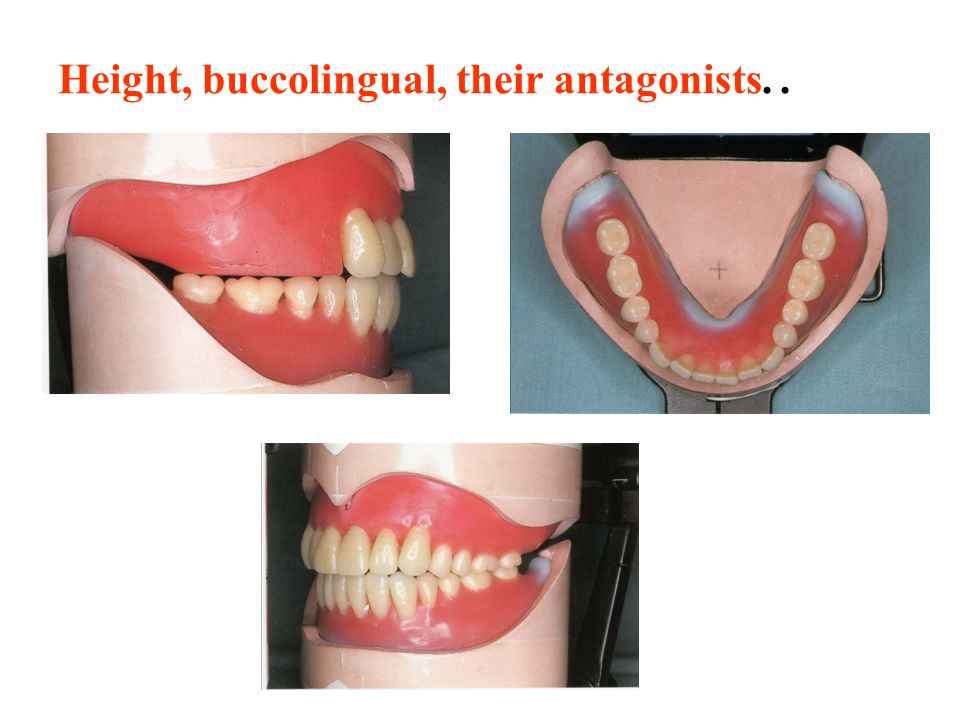This image features a detailed educational model of dentures, likely intended for instructing dental practitioners. The photograph is composed of three distinct shots: a right-side profile view displaying the lateral aspect of the teeth, a top-down view highlighting the lower row of teeth, and a three-quarter left-side profile encompassing both the upper and lower teeth. The teeth, slightly discolored, are embedded in a vivid pink and red gum simulation set into a light pink plastic base. Each vignette is set against a stark white background. Prominently visible across the images is text in red reading "Height, Bucolingual, Their Antagonists." The arrangement includes two images positioned side by side at the top, with the third image situated beneath them, giving a dispersed layout suitable for an educational context, potentially aiding trainee dental hygienists or dentists.